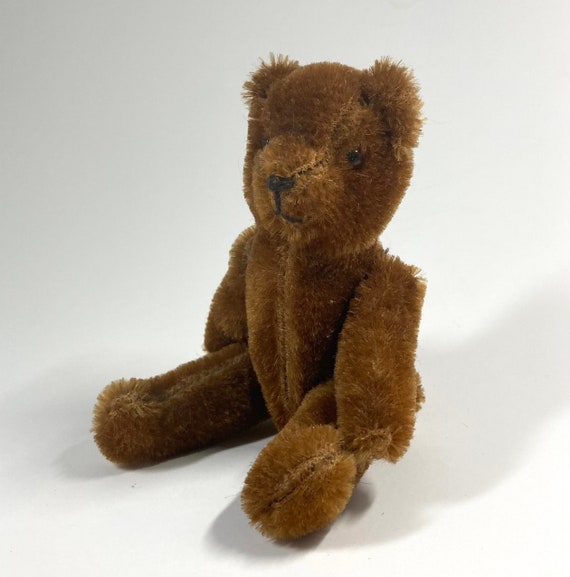In the image, there is an old, vintage brown teddy bear sitting on a white background, possibly within a light box. The teddy bear has well-worn, prickly fur, indicative of its age and use. Its color ranges from light to dark chocolate brown. The bear has two small black beaded eyes, a stitched black nose, and a stitched mouth. There are visible large stitch marks down the center of its face, torso, and legs, suggesting multiple repairs over time. The bear’s arms rest by its sides while the legs are outstretched. The lighting from the upper right casts a soft shadow, emphasizing the worn details. The bear’s ears are small and tufted like pom-poms. The overall appearance gives a sense of nostalgia and character, capturing the essence of a cherished, long-loved toy.